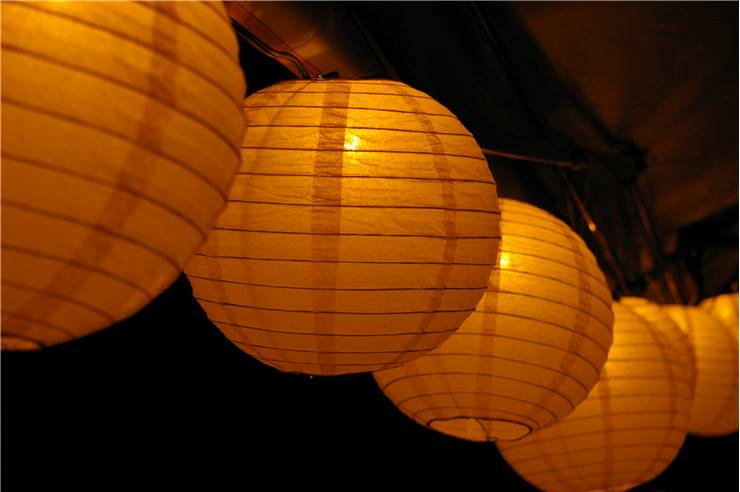Against a very dark, almost black background possibly indicative of nighttime, the image showcases a row of large, circular Chinese paper lanterns, each illuminated from within by electric lights, casting a soft yellowish-orange glow. These lanterns hang in a single file line, their arrangement suggesting they are secured by wires or clips, potentially under a wooden ceiling. The lanterns display a pattern of horizontal and vertical lines on their surfaces. The exact setting—whether it is inside or outside—is ambiguous, but the overall effect is an enchanting display of glowing lanterns in the darkness.